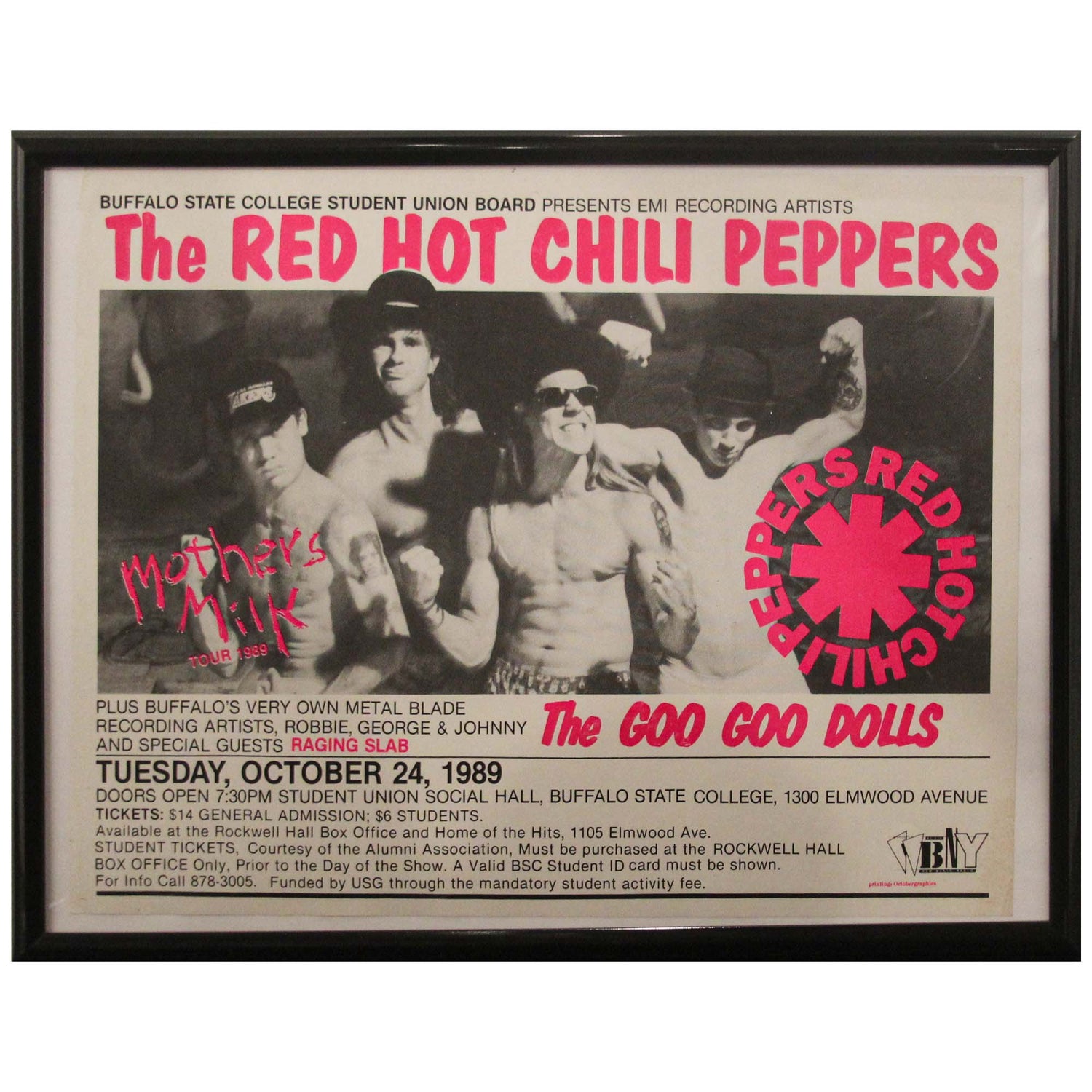This image depicts a vintage concert poster for the Red Hot Chili Peppers' "Mother's Milk Tour" dated Tuesday, October 24th, 1989. At the top, bold red text reads "Buffalo State College Student Union Board Presents EMI Recording Artists The Red Hot Chili Peppers." The central black and white photograph features four shirtless male band members, all wearing black hats, with one sporting sunglasses. To the left of the image, in red, it states "Mother's Milk Tour 1989," while to the right, the iconic Red Hot Chili Peppers asterisk logo is displayed. Additional text highlights supporting artists, including Buffalo's own Metal Blade Recording Artist Robbie, George, and Johnny, and special guest Raging Slab. The Goo Goo Dolls are also listed as performers. The event details are specified: doors open at 7.30pm at the Student Union Social Hall, Buffalo State College, 1300 Elmwood Avenue. Ticket prices are $14.00 for general admission and $6.00 for students, available at the Rockwell Hall box office and Home of the Hits at 1105 Elmwood Avenue. It notes that student tickets, courtesy of the Alumni Association, must be purchased at Rockwell Hall box office with a valid BSC student ID. For more information, it provides a contact number, stating the event is funded by the USG through a mandatory student activity fee.